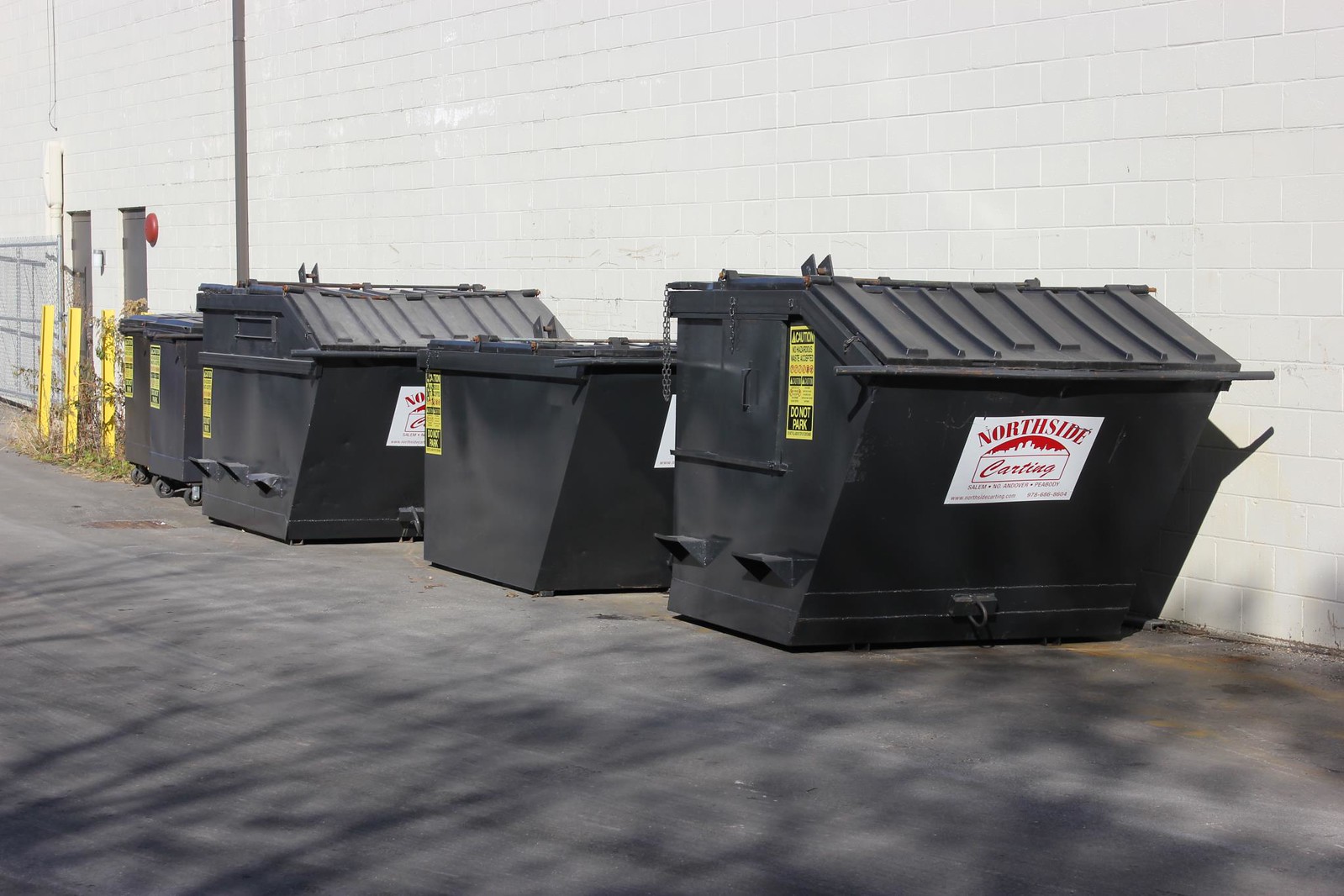In this outdoor landscape photograph, the scene is set at the back of an office or store, characterized by a large, bright white brick wall. Against this backdrop, there are four commercial-style, black metal garbage dumpsters aligned neatly on a gray pavement. They are arranged in an alternating pattern: a smaller dumpster, a larger one, another smaller one, and finally, a larger one. Each dumpster features a white label with red writing, prominently displaying the branding "Northside Cartage" along with the locations Salem, Andover, and Peabody, indicating its connection to the Boston area. Additionally, there is a website, northsidecartage.com, and a contact number, 976-686-8604, displayed on the stickers.

In the foreground, one can see a scattering of dirt in front of the first dumpster. All the dumpsters have lids designed to prevent animals from accessing the contents. Individual yellow caution signs with black writing are affixed to the sides, possibly indicating hazardous materials. The scene is completed by three vertical yellow dividers embedded in the pavement, which might be protecting a fire hydrant or related safety equipment, casting distinct shadows. Two gray doors on the white brick wall provide a utilitarian backdrop, adding to the organized and functional aesthetic of the scene.